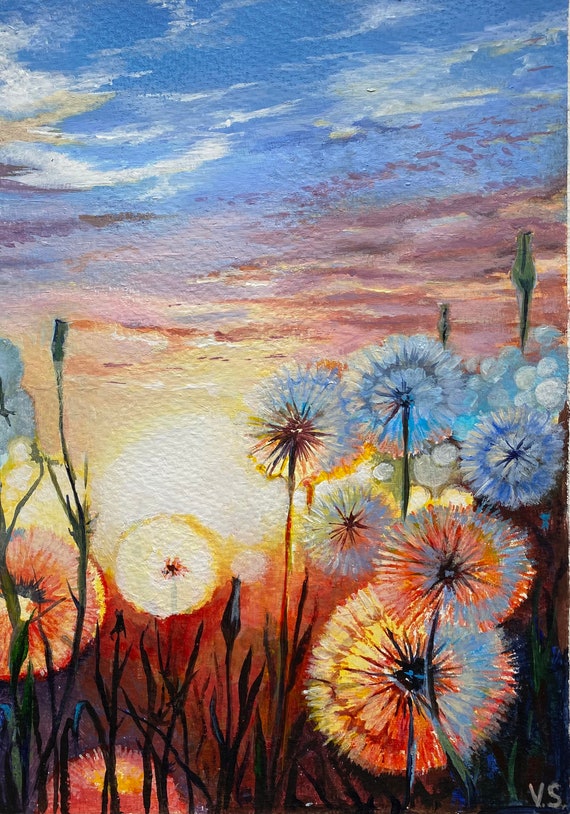This captivating oil painting, signed "V.S." in the bottom right corner, presents a mesmerizing nature scene set against a brilliant sky. The artwork, characterized by its vertical orientation, depicts a field filled with ethereal dandelion puffballs illuminated by a vivid sunset. In the foreground, approximately ten dandelions rise from thin, shadowed stems, their seed heads appearing in various hues—ranging from bright yellows and radiant oranges to soft blues and traditional greens, some yet to sprout. The light from the setting sun in the background bathes the dandelions in a warm glow, turning many of them a striking red or orange. The sky itself is a canvas of colors: a gradient of blue, orange, purple, and pink, dotted with clouds that mirror these vivid tones. The serene scene captures the transitionary moment of sunset, emphasizing the natural beauty through the delicate interplay of light and color on the canvas.